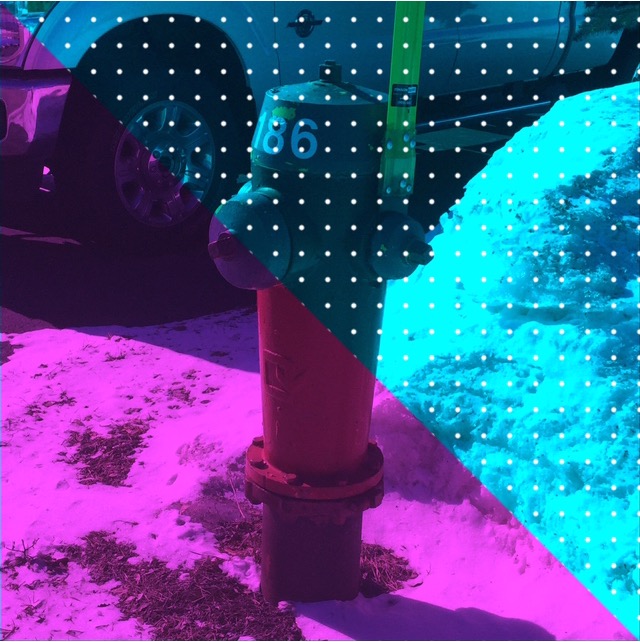The photograph features a fire hydrant in a snowy setting, partially obscured by a large pile of snow to its right, with additional snow scattered across the ground. The hydrant, identified by the number 186 painted on its cap, appears to have originally been red but is now tinted in bluish-purple hues. The backdrop includes a partially visible vehicle, possibly a white car or semi-truck, with just the tire and door visible. Graphical elements overlay the image, creating a striking visual effect: a diagonal line cuts from the upper left to the lower right, dividing the photo into two distinct sections. The left side is dominated by a vibrant magenta tint, while the right side features a cyan overlay with a pattern of tiny white polka dots. The magenta section of the image includes more of the snow pile, almost reaching the height of the hydrant itself.